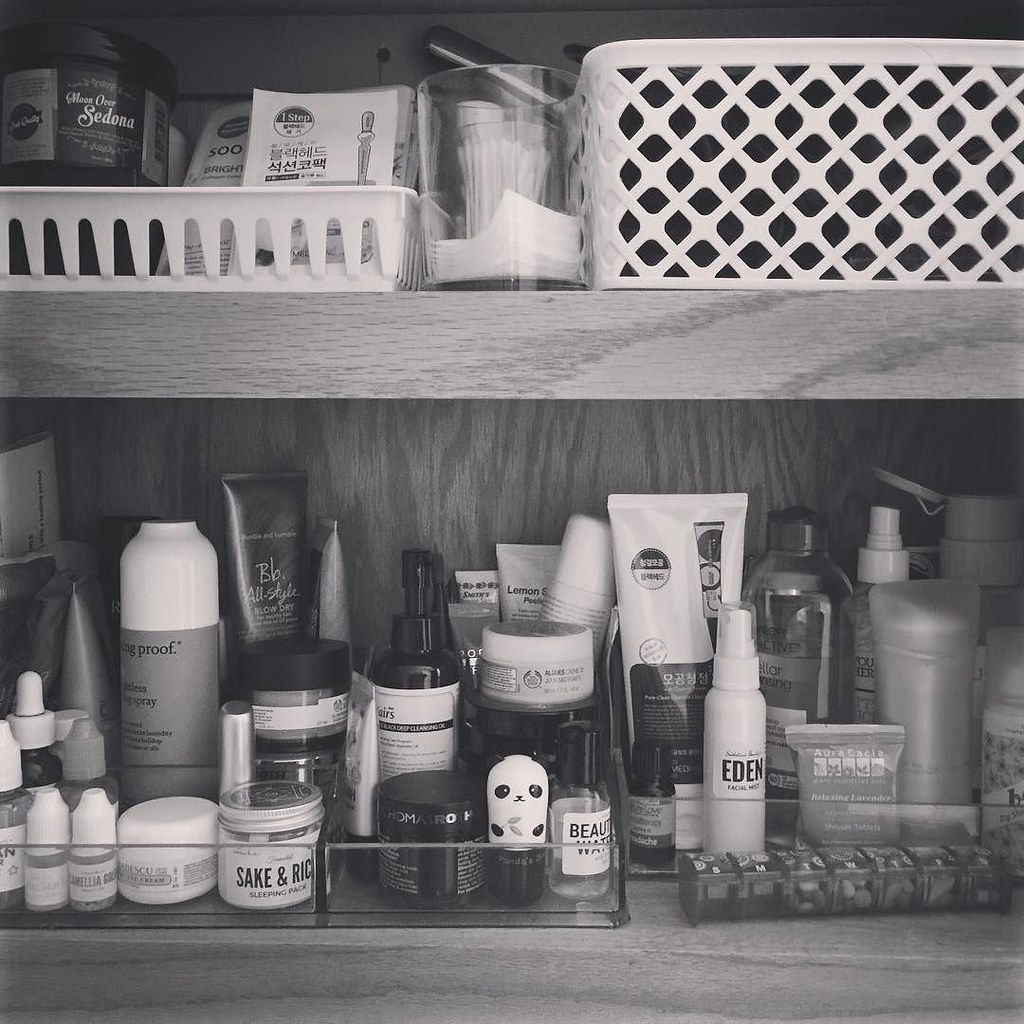A black and white photograph captures the interior of a wooden bathroom cupboard with two shelves. The wood grain on the shelves runs horizontally, while the grain on the plywood back panel runs vertically, particularly noticeable between the two shelves. On the bottom shelf, clear, short acrylic boxes organize various bottles and tubes. To the far right, a smaller bottle labeled "sack and rice" sits prominently in front. Beside it are eye drop bottles, medicine drop bottles, and a taller bottle labeled "proof," among other glass bottles and tubes. Brands and labels such as "Bibb," "blow dry," and an unlabeled item marked just with "lemon" populate the containers.

In the container next door, black containers and a panda-themed container appear, along with a clear bottle of "beauty water" bearing a white label and black top. The assortment also includes several bottles and tubes of varying heights. A pill container labeled with days of the week (S, M, T, W) sits in front, followed by another acrylic container housing additional bottles and tubes. A white bottle reading "Eden Facial Wipe" is visible amidst tubes marked with Japanese characters.

On the upper shelf, centered, lies a clear acrylic cup filled with moisture squares for makeup removal. Just behind it, another clear glass container holds Q-tips. To the right, a white basket featuring archway-like designs contains various bottles and ice packs labeled "500 bright light." Adjacent to this, a basket made up of dark triangles, possibly lined with cloth, holds items. Up towards the back left corner, several handles, likely for brushes, protrude, completing the meticulously organized and diverse collection within the bathroom cupboard’s confines.